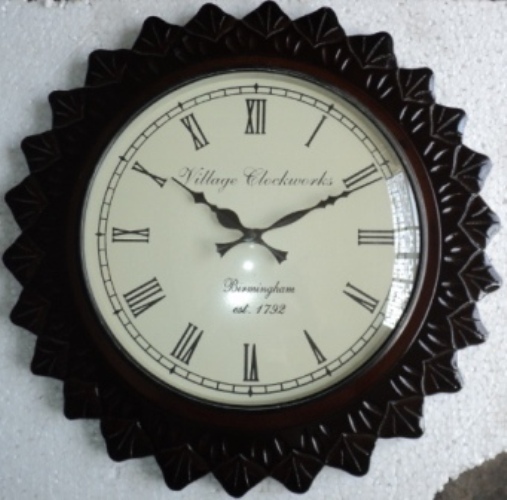A meticulously photographed antique clock rests on a plush, white pile carpet. The clock boasts a striking starburst frame made from black plastic, adorned with a series of intricate, sawtooth edges encircling its circumference. The inner clock face is a pristine white, protected by a clear, plastic dome cover. Prominently displayed across the top are the words "Village Clock Works," while underneath the central axis, above the numeral 6, it reads "Birmingham, Established 1792." The clock face is detailed with black inked numerals and railroad track markings around its perimeter, complementing the ornate black minute and hour hands. These hands feature distinct triangular tips and bulged segments pointing towards the numbers. The time shown on the clock is precisely 11 minutes past 10 o'clock.